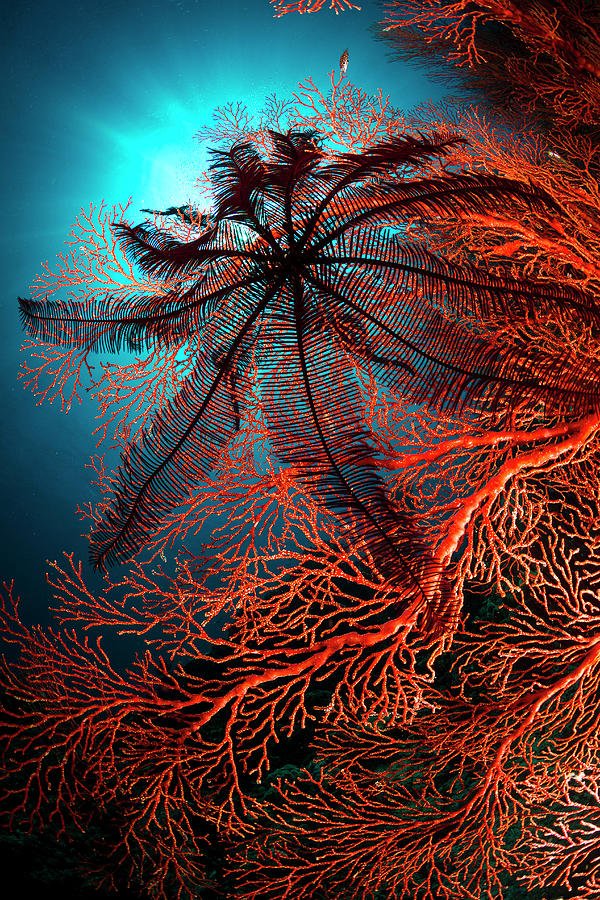This captivating underwater photograph showcases a vibrant, tree-like coral formation stretching from the right side of the image to the left. The coral appears in striking orange and red hues, resembling the intricate branching structure of bronchioles or fine tree limbs, with thick bases gradually tapering into thinner branches. Interwoven with this vivid coral is a silhouetted black shape, reminiscent of a starfish or the fronds of a fern. The image captures the coral scene from below, looking up toward the surface, allowing the blue background and a bright light source—likely the sunlight filtering through the water—to illuminate the delicate beauty of this underwater wonder.